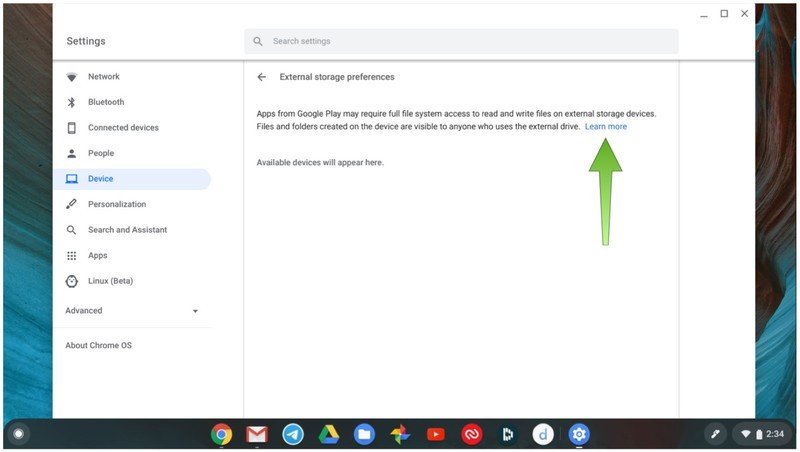This image is a detailed screenshot of a desktop, specifically showcasing the settings menu within a Chrome OS environment. The interface is set against a clean, white background. On the left side of the screen, there is a vertical navigation panel titled "Settings" in small, black letters at the top. This panel lists various setting categories in the following order: Network, Bluetooth, Connected Devices, People, Device, Personalization, Search and Assistant, Apps, Linux (Beta), Advanced, and About Chrome OS.

On the right side of the screen, there is a detailed settings page titled "External Storage Preferences," indicated by a header at the top with a left-pointing arrow for navigation. The text beneath this header explains that apps from Google Play may require full file system access to read and write files on external storage devices. It also notes that files and folders created on the device are accessible to anyone using the external drive. There is a "Learn More" hyperlink below this explanatory text, accompanied by a green arrow edited into the image, directing attention towards the hyperlink.

At the bottom of the screenshot, the screen taskbar is visible, displaying a set of frequently used applications: Google, Gmail, YouTube, Settings, and others, all centrally aligned for easy access.